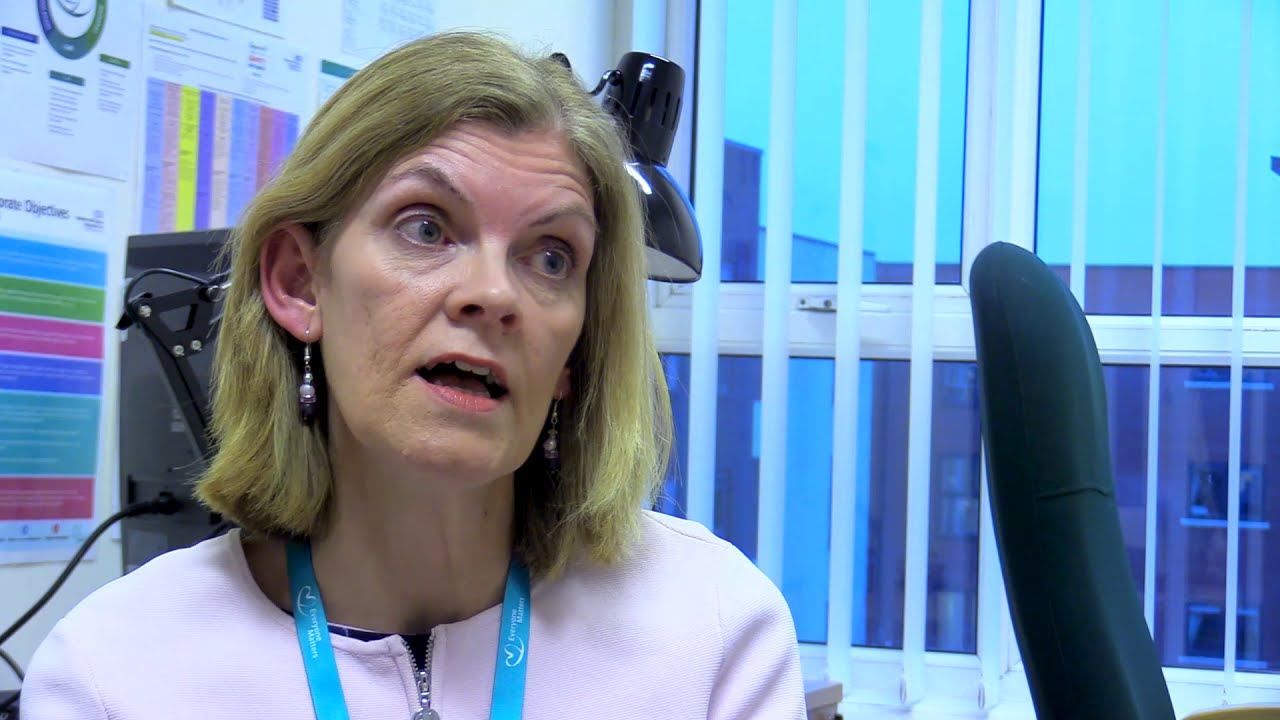In this professional-looking photograph, a woman in her fifties, with short blonde shoulder-length hair and earrings, appears to be speaking or being interviewed. She wears a light pink or white jacket and a light blue lanyard, likely holding an ID tag, around her neck. The scene resembles an office setting, featuring a black lamp behind her and an adjacent window with unobstructed shades revealing a tall building and the sky outside. The wall behind her is adorned with various charts and pieces of paper, suggesting an informative environment. She sits in or near a black or gray chair, and the overall composition suggests the photo was taken during a news segment or documentary interview, underscoring the professional tone of the image.